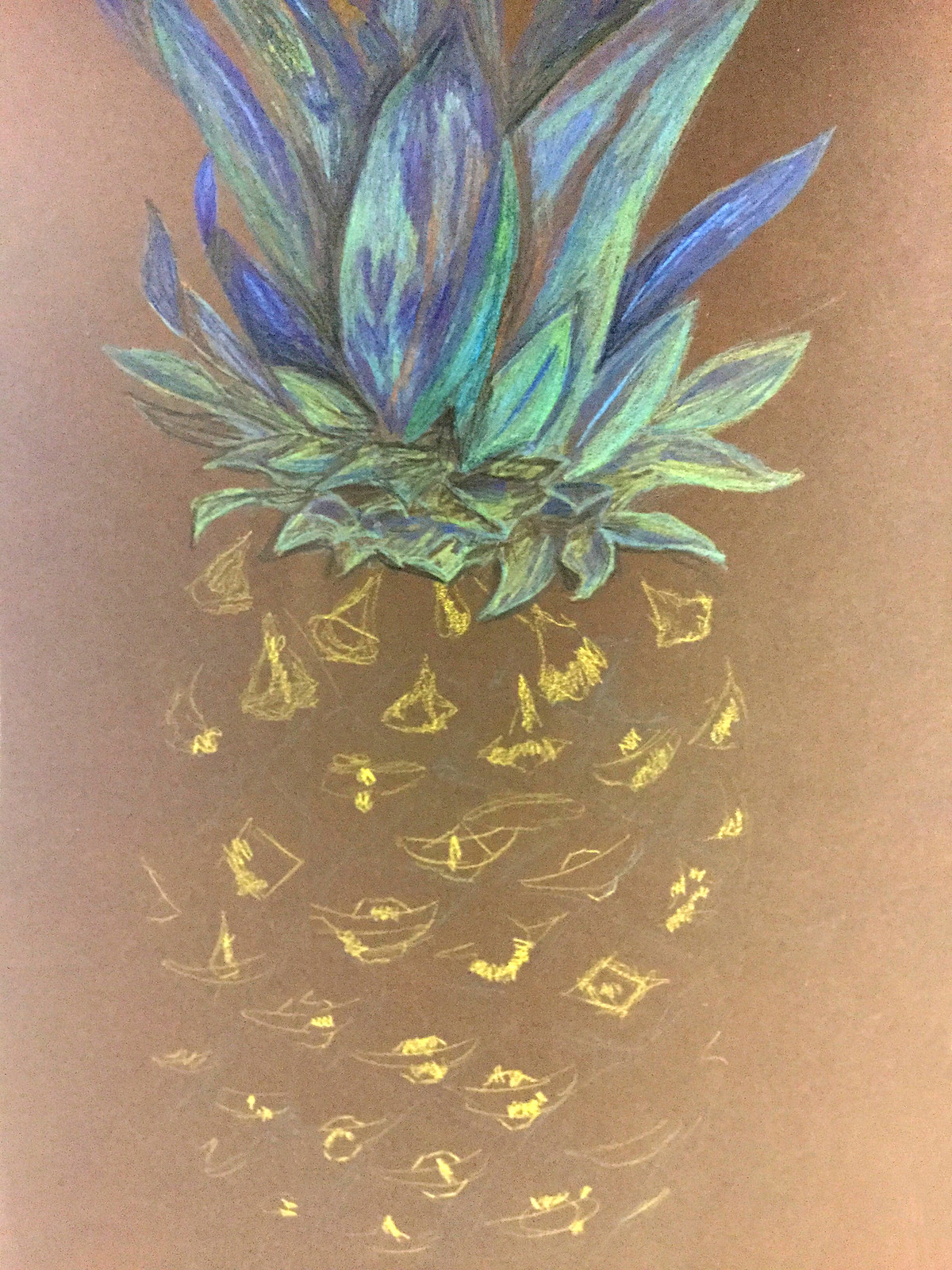This image showcases a vibrant artwork of a pineapple, drawn with colored pencils on a brown construction paper background. The pineapple dominates the image and lacks a traditional outline, its shape instead formed by yellow, triangular highlights filling in the fruity texture. There's a faint white-gray border subtly cutting around these triangles. At the top, the pineapple's leaves are depicted in an eclectic mix of neon blue and darker blue, with smaller, neon teal and green leaves at the base, transitioning to larger, bluish-hued leaves towards the top. The artwork blends colors creatively, with possible signs of chalk or paint enhancing the texture. The background features a smoky black or gray shade, adding contrast to the colorful pineapple. This detailed, vibrant drawing has a unique, homey appeal, perfect for display.